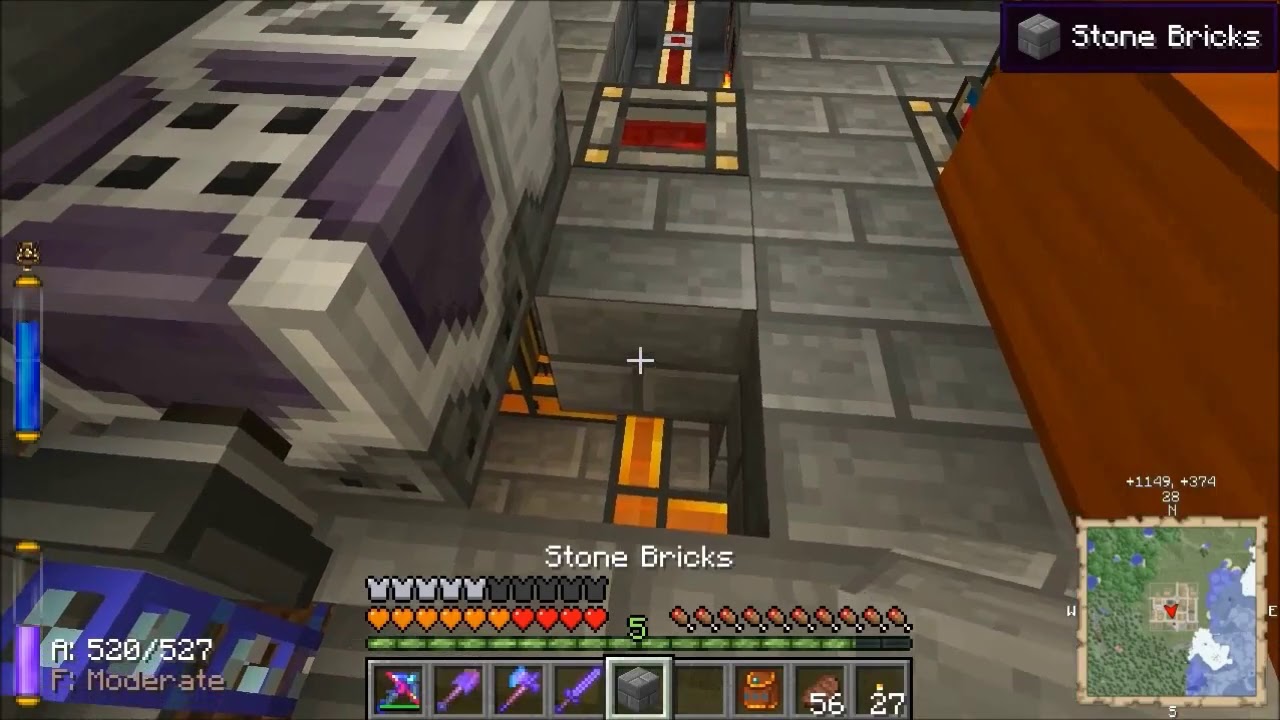This detailed screen capture from the game Minecraft highlights a pixelated, blocky aesthetic reminiscent of early Nintendo games. The bottom of the screen features an extensive toolbar spanning eight slots, stocked with various items such as shovels, axes, and swords, each marked with numerical quantities. Above this toolbar, player health is indicated by colorful heart icons, and additional stats and meters, including a half-depleted body armor bar and a green bar with tic-tac markers, clutter the left sidebar.

The image showcases a scene where the player appears to be modifying the structure of a building, evident from the visible demolition and crafting. The lower right corner houses a mini-map with terrain details and coordinates, aiding navigation. Bricks in purple and gray hues, aligning with potential netherstone and regular stone bricks, protrude on the left, suggesting an immersive in-game construction. On the right, an extending medium brown pillar, mimicking wood, contrasts the other materials. Centered within the image are varied bricks, with colors ranging from gray to orange and red, indicating a complex layered composition. Notably, the top right corner displays "stone bricks" accompanied by a gray block icon, reinforcing the game's crafting and building theme.